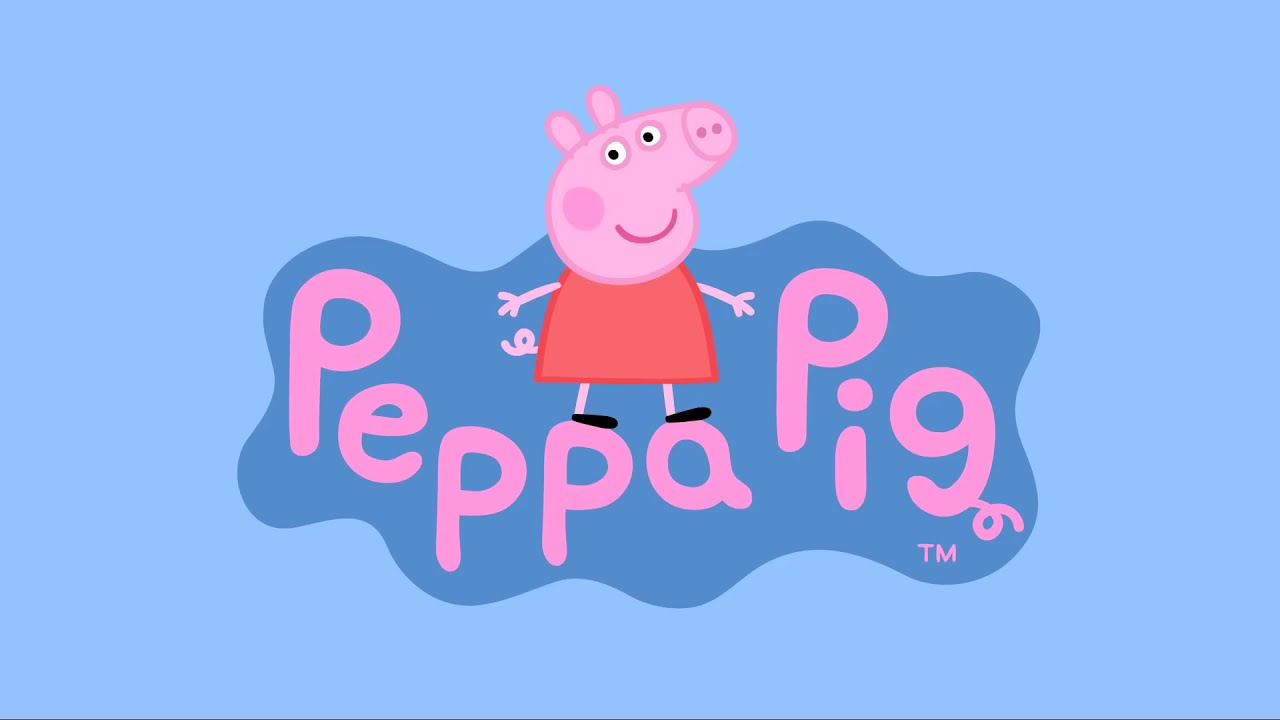The image is a rectangular title screen for the cartoon show Peppa Pig, characterized by a playful and vibrant design. It features a light blue background with a dark blue, wavy, cloud-shaped blob at the center. The name "Peppa Pig" is prominently displayed in pink letters, with "P-E-P-P-A" on the top and "P-I-G" below, where the final "G" has a coiled tail attached. There is also a trademark symbol (TM) next to the word "Pig."

Peppa Pig, the cartoon character, is standing atop the letters "P" and "A" of "Peppa," presenting herself with a wide, friendly smile. She has a pink body, googly eyes, a snout, a red mouth, and a distinctive pink cheek spot. Peppa is wearing a red dress and black shoes, with her simple, cartoon-styled arms extended outward, each ending in three fingers. Her overall design is stylized to appear easy and approachable, resembling artwork a child might create with construction paper. The color palette includes various shades of pink for Peppa and the lettering, maintaining consistency and making the character the centerpiece against the soothing blue background.